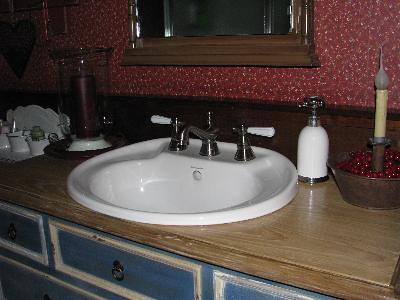In this color photograph, a bathroom sink is the focal point. The wall behind the sink features vibrant red wallpaper adorned with a delicate pattern of white flowers. A mirror with a dark wooden frame hangs above the sink, reflecting elements of the room. To the left of the sink, a dark-colored pillar candle resides in a glass container, accompanied by several small white porcelain pots. The white basin is complemented by matching white handles and a silver faucet. To the right of the basin, a white pump bottle sits alongside a glass bowl filled with red spherical objects, from which an electric candle protrudes. The sink’s wooden-colored counter stands in contrast to the blue and white painted area below it. The photograph contains no legible writing, people, animals, plants, flowers, trees, or motorized vehicles.